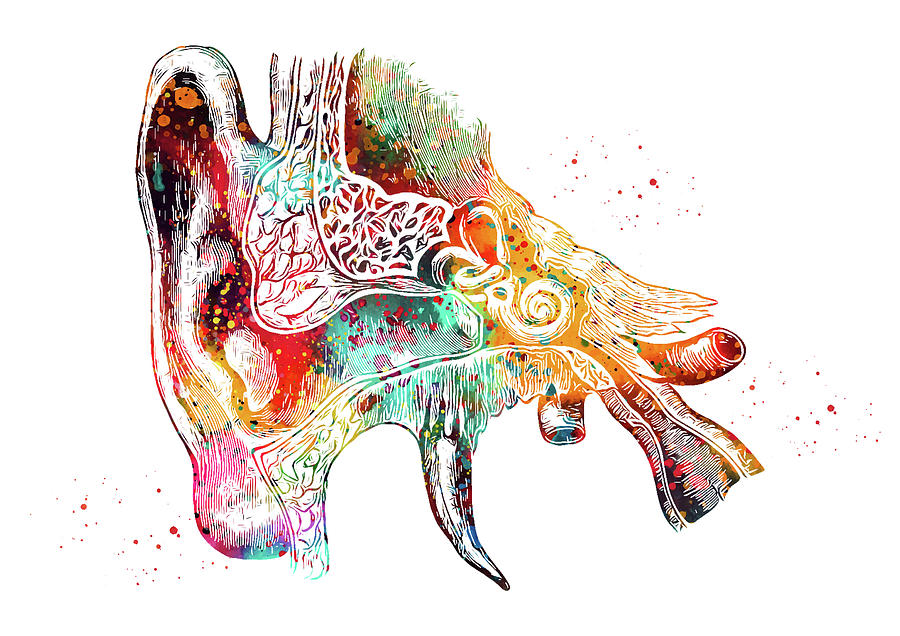The image is a vibrant, abstract illustration featuring what seems to be an ear or perhaps another human organ, given its anatomical details. The object is vividly painted in an array of colors including shades of pink, red, green, yellow, orange, and mint green. It appears wrapped in something, with a distinctive horn-like part on the bottom, adding to its curious shape.

On closer inspection, the painting also appears to integrate other anatomical features like the ear canal and possibly even arteries, though their scientific accuracy is uncertain. The entire composition is speckled with multicolored dots, predominantly magenta, contributing to a polka-dotted appearance. There are noticeable splatters of red paint on both the bottom left and right sides, resembling a paintbrush effect.

The background remains white, making the colorful subject stand out strikingly. The overall effect is a mesmerizing, complex blend of anatomical and abstract elements, unified by a rich palette of bright hues and artistic splatters.